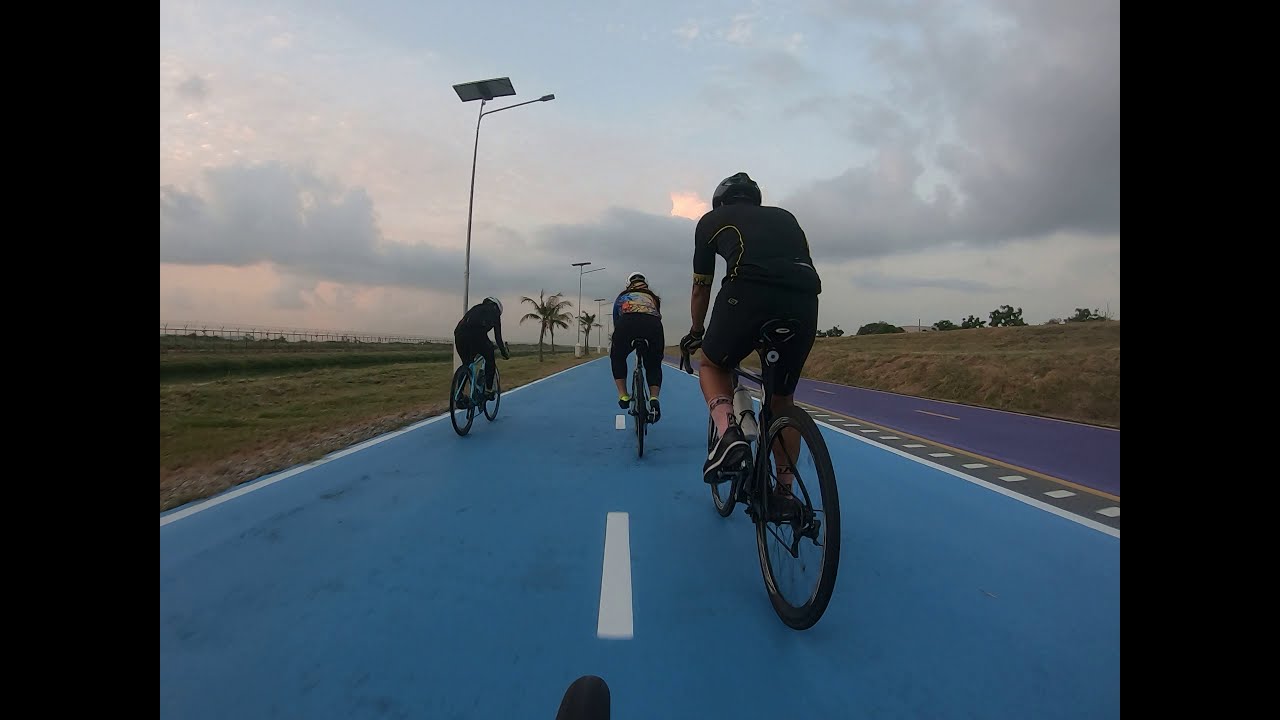This photograph captures three cyclists from behind as they ride away on a smooth, dark blue road, delineated with a central dashed white line and solid white side lines. The cyclists and their bikes predominantly feature black attire and equipment: the closest cyclist, positioned just right of the center line, wears an all-black outfit including their helmet, shoes, and bicycle, with only a small white section near the handlebars. The cyclist in the center sports a more colorful outfit with a rainbow-colored shirt, black shorts, and a light-colored helmet. The cyclist on the left is dressed in all black with a whitish helmet and rides near the solid white line. The scene is set in the countryside, framed on either side by low grass and palm trees. To the right of the blue road is a purple road marked by solid yellow lines on the edges and a dashed yellow line in the center. Additional details include vertical black bars along the left and right edges of the photograph, street lamps stretching into the sky, and a hazy blue sky with dark clouds, suggesting the time is either early morning or near dusk.